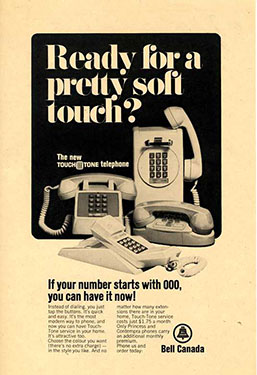The image is an old advertisement, likely from the late 70s or early 80s, featuring a promotional flyer from Bell Canada for their new touch-tone telephones. The ad, printed on yellowish-brown paper that appears aged and slightly deteriorated, displays four house phones, each designed with a button dial pad rather than the older rotary dial. These phones, depicted in black and white, are set against a lightly pinkish white rectangle background with a distinct black square highlighting the text. At the top, it reads, "Ready for a pretty soft touch" and below, "The new touch tone telephone." At the bottom of the ad, it states, "If your number starts with 000, you can have it now," followed by smaller, unreadable text and the Bell Canada logo.